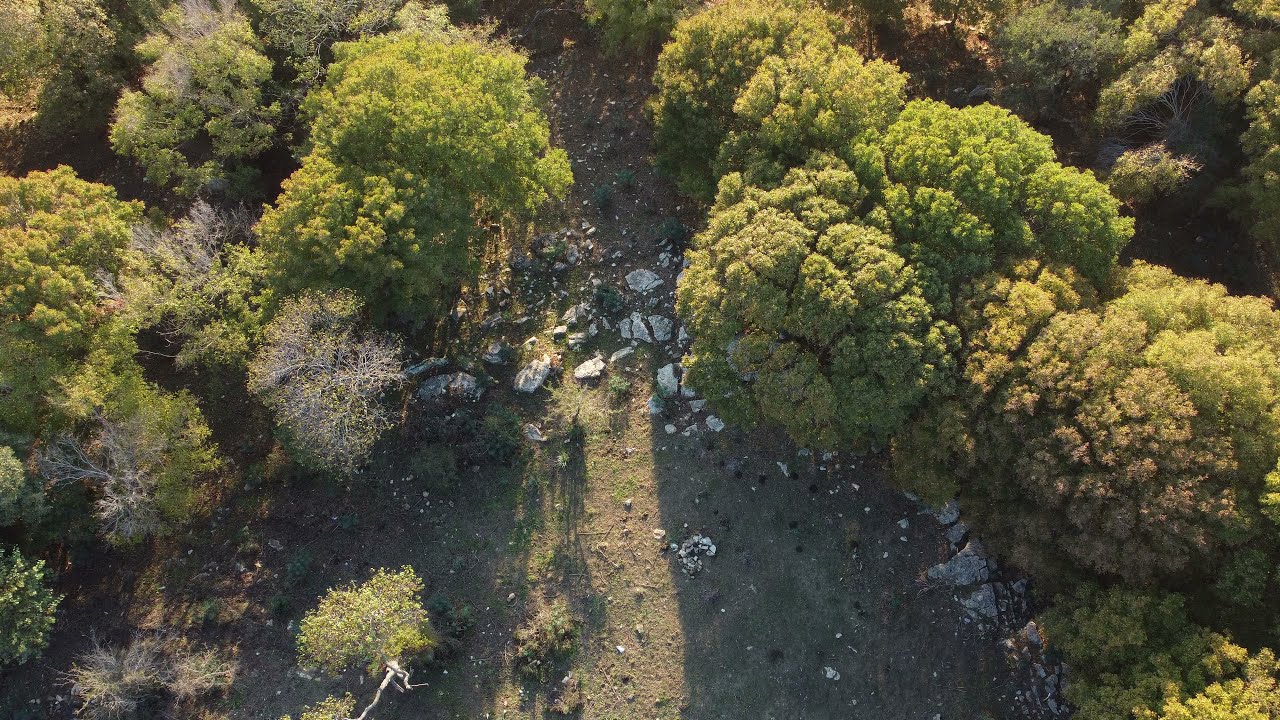This image shows an aerial view of a densely wooded area characterized by thick, bushy trees with lush foliage. The trees predominantly appear in various shades of green, from darker hues to lighter yellow-greens, with some areas almost giving off a shade like broccoli tops. Scattered throughout the image, particularly in the middle, are patches of gray rocks and other white debris, possibly crushed rock, amid a landscape of brownish-green ground mixed with dirt and grass. The image, rectangular in shape, also features darker shadows on the top right and bottom corners, giving those areas a muted green-gray ambiance. This diverse mix of elements—trees, rocks, and dirt—gives the scene an unkempt, natural appearance with visible debris and dead weeds interspersed among the vibrant foliage.